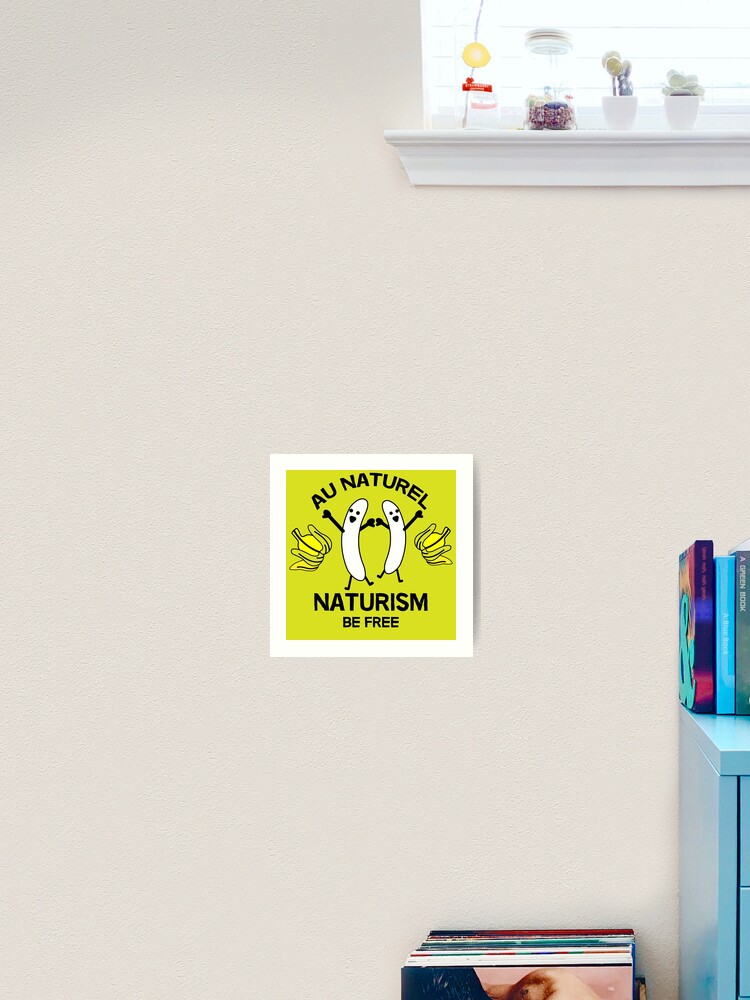The image depicts a cozy room with a modest wall adorned in beige. At the center of the wall is a small, white-edged poster with a pea-green interior. It features black lettering that reads "Ah Natural" and showcases quirky, cartoon-like figures that appear to be beans or hot dogs with black hands and feet, flanked by floral or vegetable motifs. Below this, it reads "Naturism, Be Free" in the same black font. The right side of the image captures the upper portion of a window with sunlight streaming through the blinds onto a white windowsill, which holds two plants and a mason jar containing water and some items. In the lower left corner stands a blue dresser or cabinet, topped with a few books, and adjacent to it, a neat stack of LP records is visible. The room, suffused with natural light, presents a tranquil and eclectic atmosphere, with the primary focus on the whimsical "Ah Natural, Naturism, Be Free" poster.